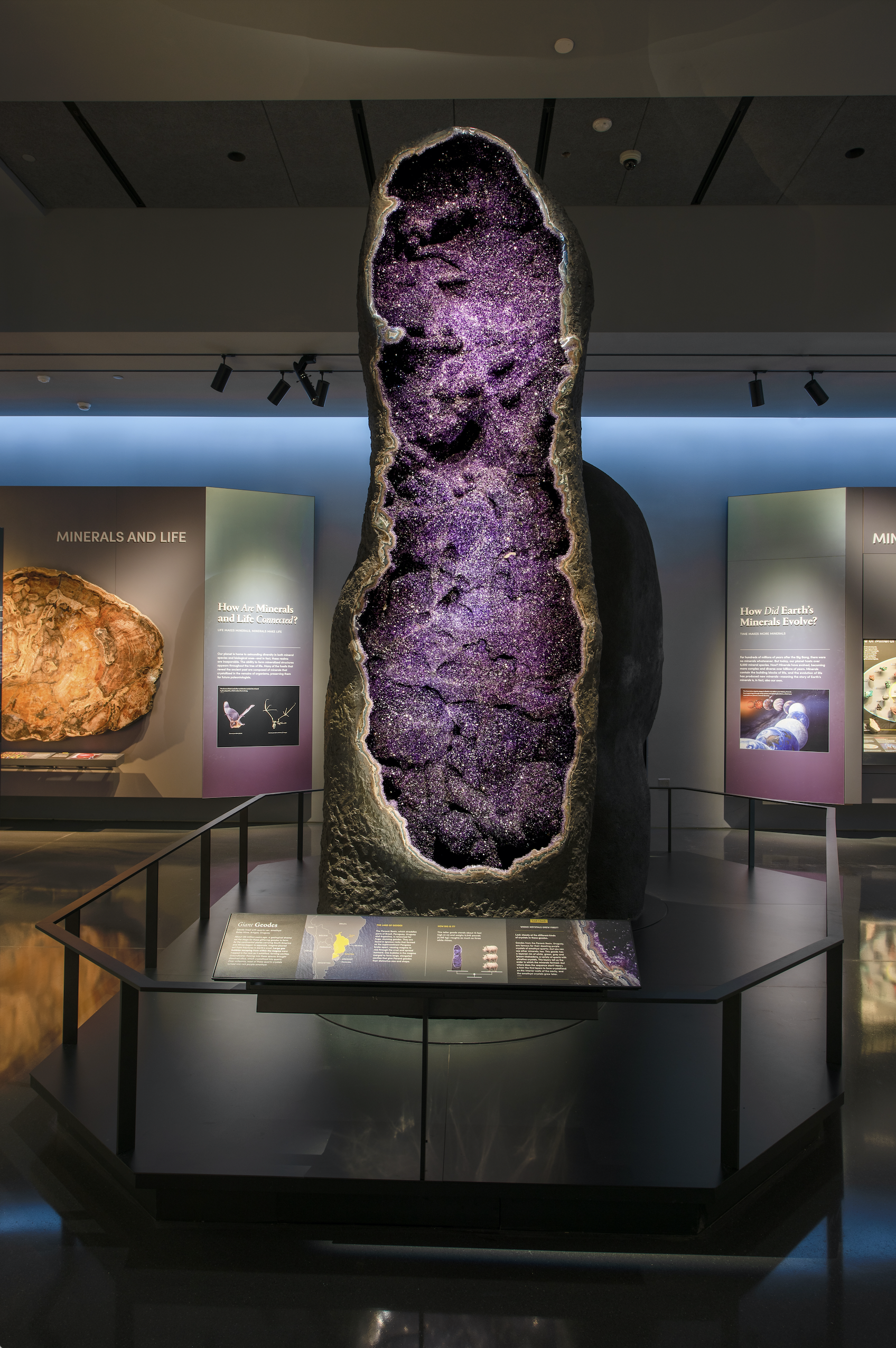The image captures an exhibit within a modern, minimalist museum featuring a strikingly large geode, estimated to be at least five to six feet tall. The display is set against a backdrop adorned with the header text "Minerals and Life," accompanied by various images and text panels about rocks and minerals, though most of the text is too small to read. The geode itself, a vertical cutout originating from the southeastern region of Africa, showcases a mesmerizing interior with deep purple hues that resemble a night sky, illuminated by numerous reflective points from the overhead track lighting. This main exhibit is enclosed by a small fence, and accompanied by a plaque detailing information about the mineral, though the text is not legible in the image.